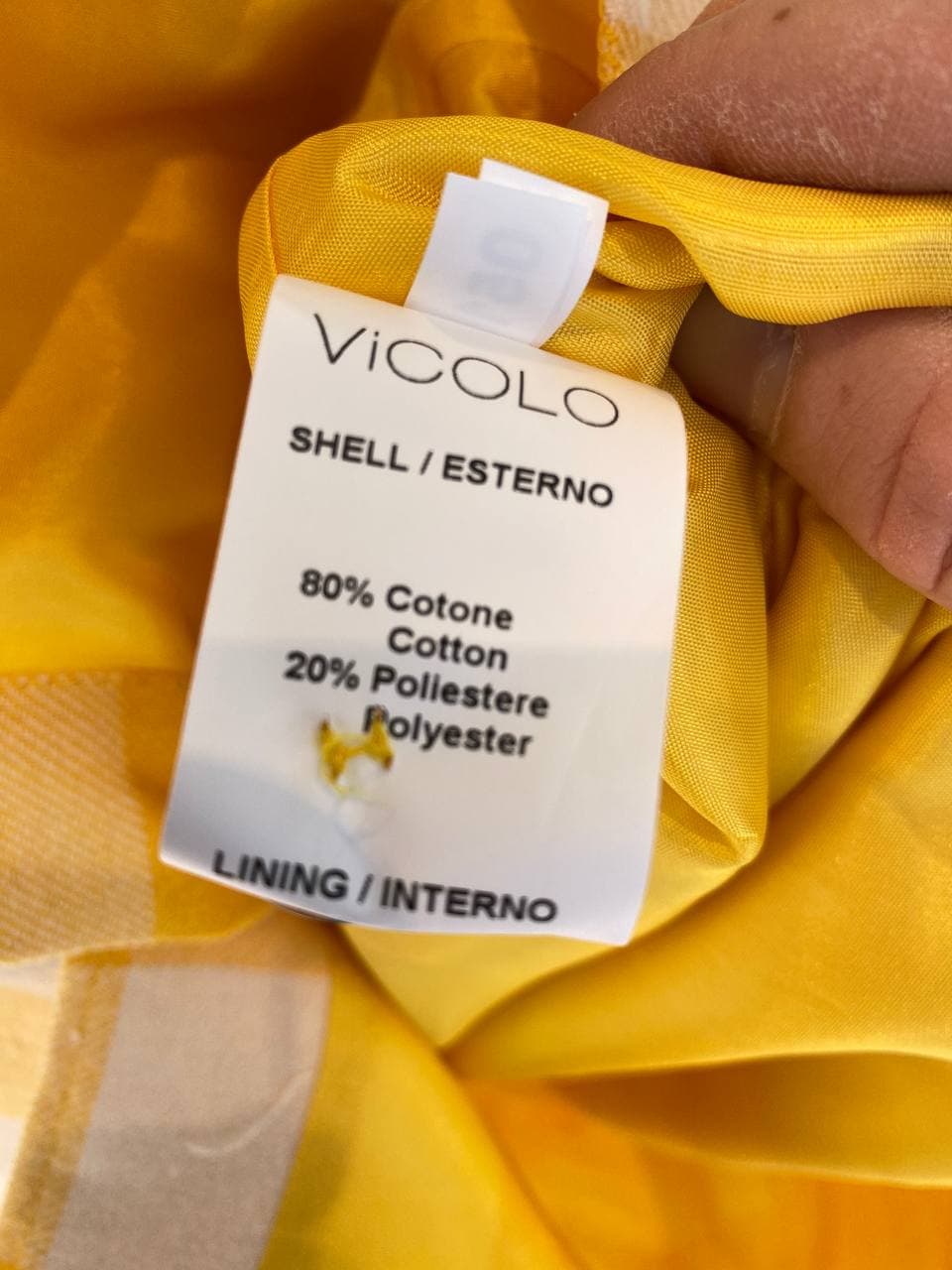This rectangular photograph, which is taller than it is wide, presents an extremely zoomed-in image of a crumpled, sheer yellow fabric, revealing intricate weave details. Dominating the center of the image is a white washing instruction tag that reads "Vicolo," under which it specifies "Shell/Esterno: 80% Cotton (Cotone), 20% Polyester (Poliestere)," followed by "Lining/Interno." The fabric appears to be a blend of cotton and polyester. In the upper-right corner, the index and thumb fingers of a Caucasian person are visible, gripping the fabric. The individual's forefinger shows noticeable dryness and peeling of the skin. The color palette of the image is primarily yellow, with touches of black, white, brown, and the skin tones of the hand. Despite the ambiguity about the fabric's actual purpose, the photograph provides a detailed, close-up view of its texture and the tag's precise information.